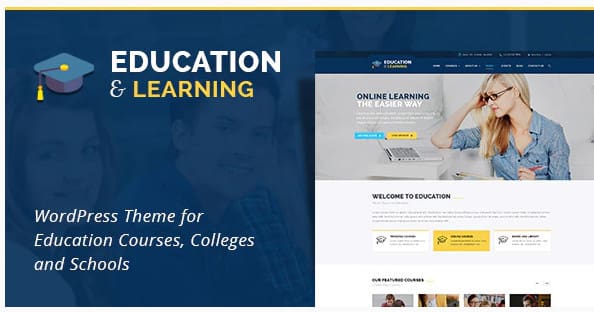A screenshot from an advertisement displayed on a computer screen. The advertisement has a navy blue background with a distinctive yellow stripe running along the top. At the top of the ad, there is a stylized graduation cap in blue and gold accompanied by the text "Education and Learning." The word "Learning" is highlighted in yellow, while "Education" and "and" are in white font.

Below this, the ad states, "WordPress theme for education courses, colleges, and schools." The main visual element features a group of young students, possibly high school or college-aged. They are smiling and looking towards the screen, shrouded slightly by the ad's dark background.

On the right section of the screenshot, a webpage is open, showing a banner that reads, "Learn Online: Learning the Easier Way." The image on the webpage features a woman with long blonde hair wearing glasses. She is holding a pen and appears to be engaged in note-taking, with a notebook and a laptop open beside her. The text "Welcome to Education" is displayed prominently.

Toward the bottom of the ad, there are three rectangular boxes in a sequence of colors: white, yellow, and white.